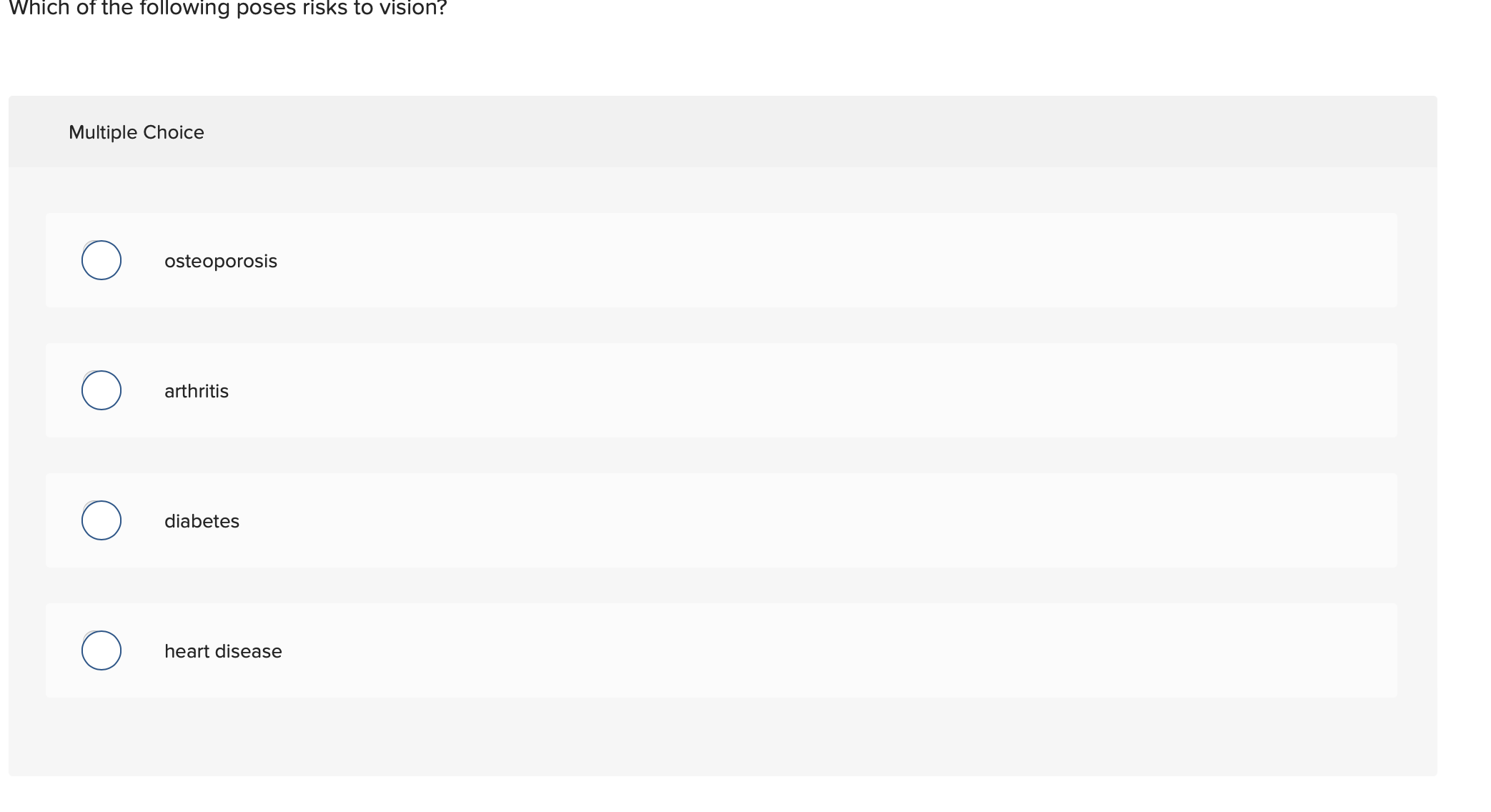The webpage segment displayed features a partially visible section of an interactive questionnaire designed to assess knowledge about vision health. The background is primarily light gray, supplemented with several off-white text boxes. The webpage design includes a series of radio buttons (bubbles) positioned to the left of each answer option.

At the top of the segment, the question posed is, "Which of the following poses risks to vision?" Below this inquiry, nestled within the light gray area bordered distinctively, the text clarifies that this is a multiple-choice question. The listed answer options, each with an accompanying bubble for selection, are:
1. Osteoporosis
2. Arthritis
3. Diabetes
4. Heart Disease

None of these options are pre-selected. The question is reiterated again, prompting the user to identify which conditions pose risks to vision. The overall design of the webpage is minimalistic, characterized by its muted color palette—light gray backgrounds with off-white accent boxes—and is simplistic, featuring clear and organized vertical alignment of the multiple-choice answers. The radio buttons beside the options are the only elements in a pure white, standing out against the subdued tones of the rest of the page.